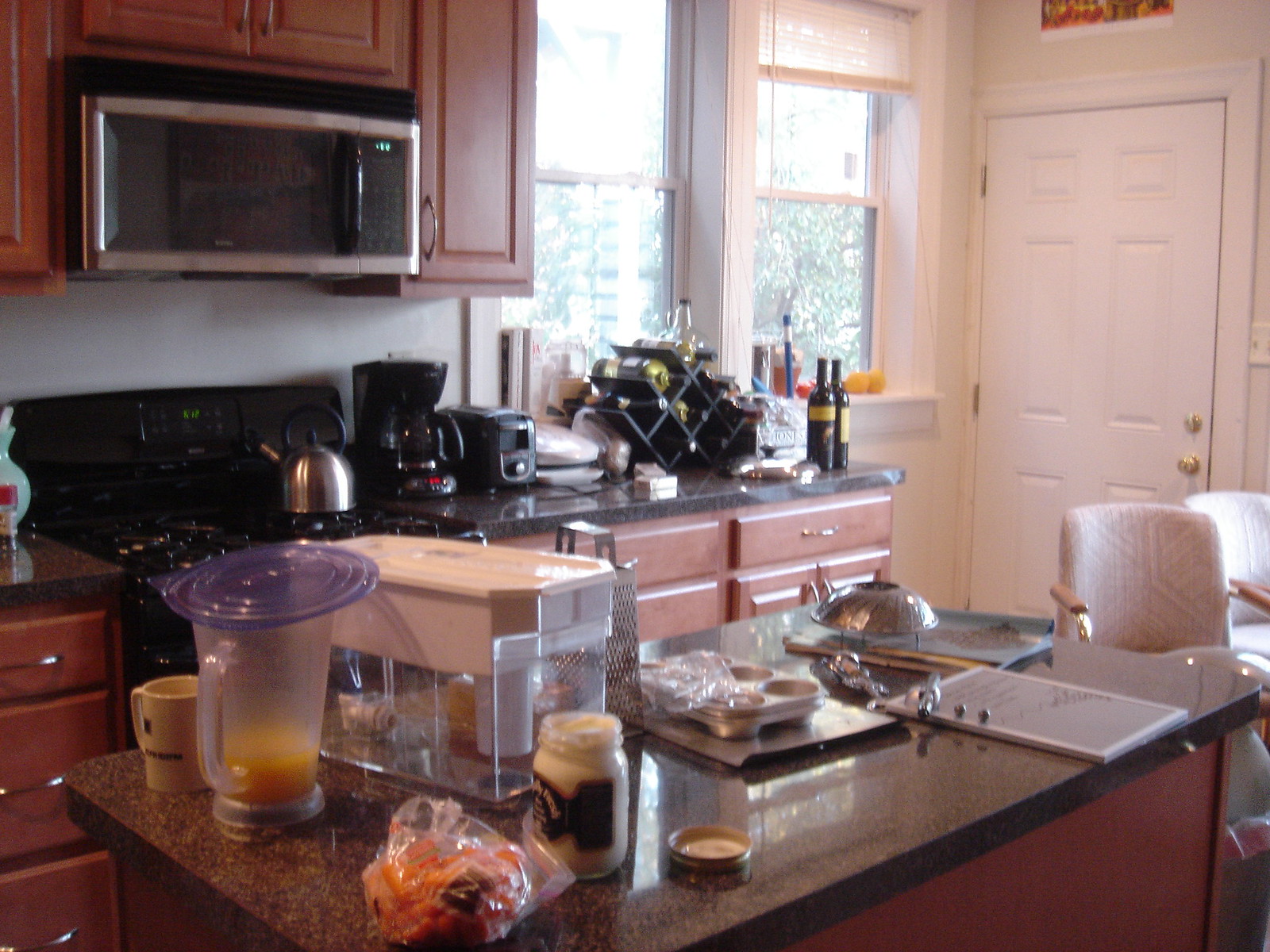The image showcases a well-appointed kitchen. In the top right corner, there is a pristine white door and door frame. To the top left, brown cabinetry features a built-in slot that houses a sleek, silver-colored microwave. Below the microwave, a black stove range is prominently displayed. On the countertop to the right of the stove sits a coffee maker, with a black toaster positioned even further to the right. A silver kettle rests on one of the stovetop burners. To the right side of the image, a black wine rack stands adjacent to several bottles of wine arranged on the counter.

In the foreground, a kitchen island serves as a central workspace. It holds a blender containing a small amount of orange juice, a plastic bag filled with carrot sticks, and a jar which appears to contain either mac and cheese or tartar sauce. Additionally, there is a large water filter stationed on the island, and a package of muffin tins positioned to the right completes the scene.

Overall, the kitchen appears well-equipped and organized, combining functional elements with an elegant aesthetic.